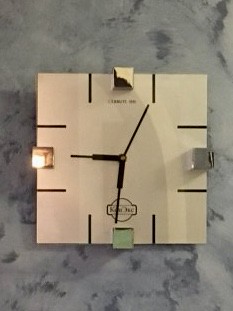This image features a square clock, elegantly mounted against a light gray marble backdrop adorned with sporadic darker gray veining. The clock itself is of a light beige or tan hue, exuding a minimalist and contemporary design. Its three hands include a thicker short hand for the hours, a longer but equally thick black hand for the minutes, and a slender, elongated hand for the seconds. The face of the clock lacks traditional numerals, opting instead for simple, understated lines approximately a couple of inches in length to mark the hours. The setting suggests that the clock could either be hanging on a wall or resting flat on the sophisticated marble surface, enhancing the overall aesthetic appeal.